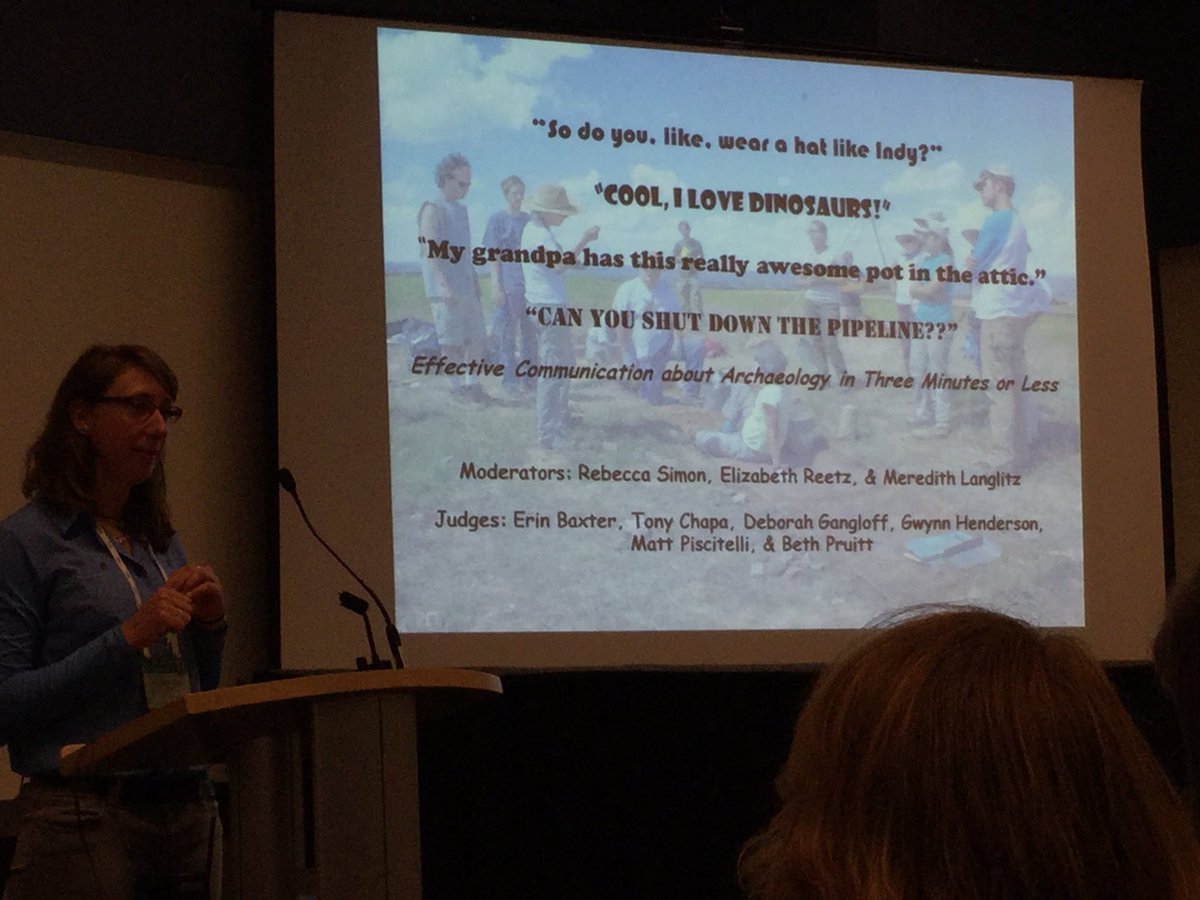In the photograph, a female presenter is delivering a talk at a conference. She stands at a lectern, where both a large and a small microphone are positioned. She's dressed in a blue button-up top and khaki pants, accessorized with a lanyard. Her brown hair and eyeglasses complete her professional appearance. Her hands are clasped together as she speaks, conveying confidence and authority.

Behind her, a projection screen is pulled down, displaying text fragments that suggest a dialogue or brainstorming session on the theme of effective communication in archeology. Phrases like "so do you, like, wear a hat like Indy," "I love dinosaurs," "my grandpa has this really awesome pot in the attic," and "can you shut down the pipeline??" appear on the screen, followed by the title "Effective communication about archeology in three minutes or less."

Additionally, the names of the session's moderators—Rebecca Simon, Elizabeth Rietz, and Meredith Langates—as well as the judges—Erin Baxter, Tony Chapa, Deborah Gangloff, Quinn Henderson, Matt Machete, and Beth Pruitt—are listed. In the foreground, the heads of audience members are visible, indicating that the presentation is well-attended.